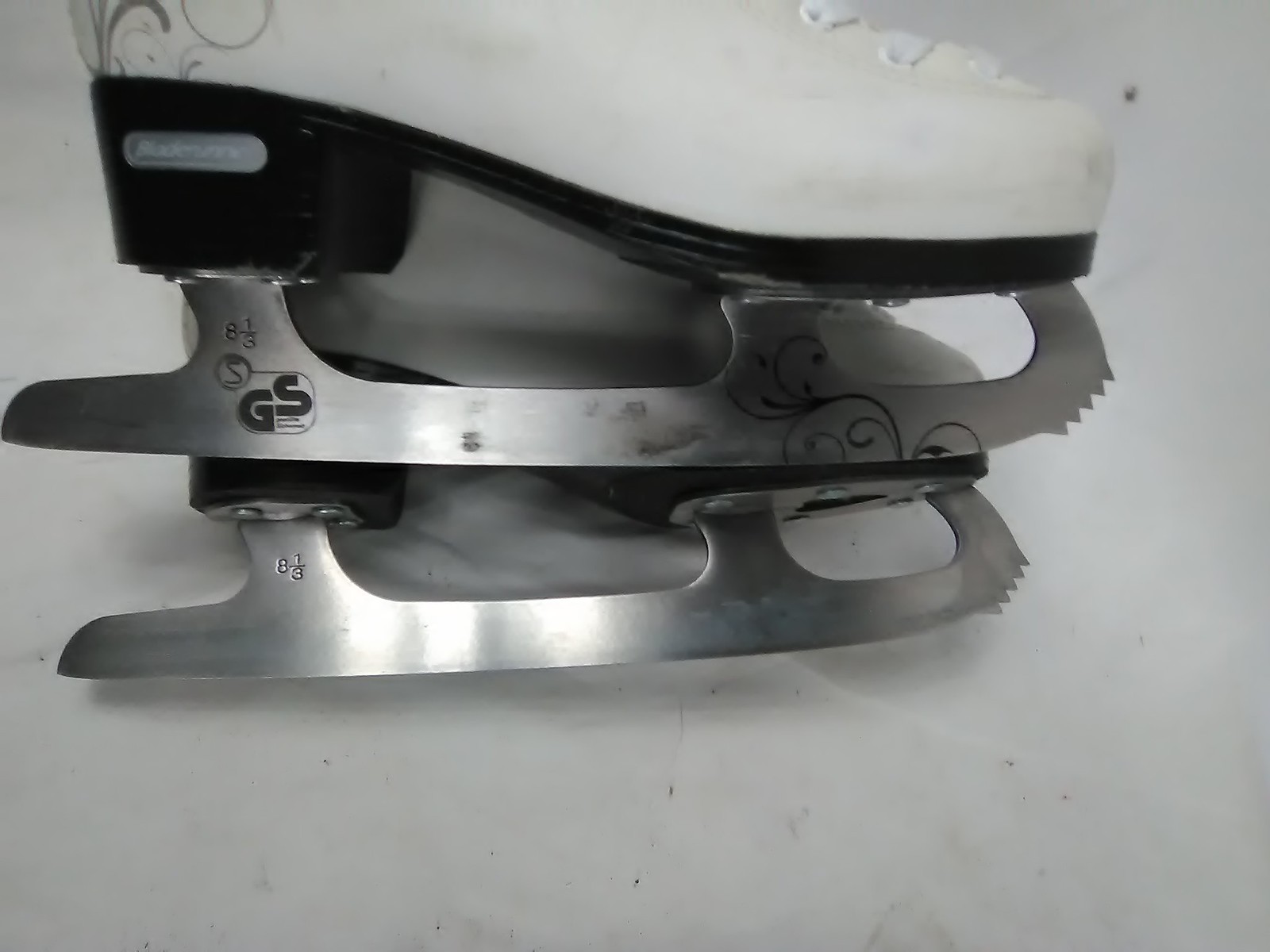This detailed black and white photograph captures a pair of white ice skates with black heels and soles, set against a light, possibly icy or white background. The skates are positioned such that one skate is prominently in the foreground, while the other is partially obscured behind it. The image is taken from a low angle, emphasizing the gleaming silver blades which reflect the light, highlighting their intricate design. The skates have white laces visible at the top, and each blade is etched with the size "8 and 1/3." Additionally, the initials "GS" appear on the black back of one skate and on the blade, accompanied by a matching floral or leaf pattern in gray on the heel area. The close-up nature of the photograph, focused on the blades, brings attention to these detailed elements, including the design and the specific markings.